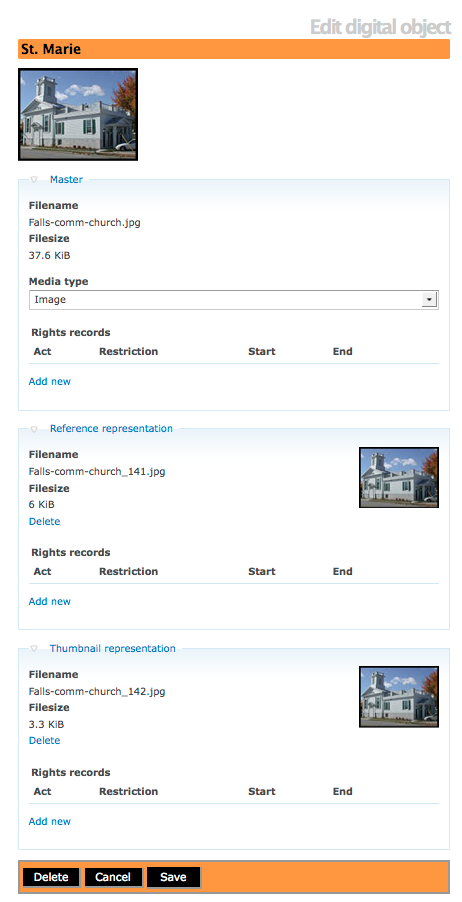The image showcases a digital editing interface for an image titled "Sainte-Marie Church." The interface provides extensive details about the image files such as file name, size, type, and access restrictions. The original image, displayed prominently, is named "falls-com-church.jpg" and has a file size of 37.6 kilobytes. Below it, two additional representations of the image are shown as thumbnails. The second image, named "falls-com-church_141.jpg," is slightly smaller at 6 kilobytes. The third image, labeled "falls-com-church_142.jpg," is the smallest at 3.3 kilobytes. The arrangement of the images from largest to smallest provides a clear view of the different file sizes and names, indicating varying resolutions or versions of the original "Sainte-Marie Church" image.